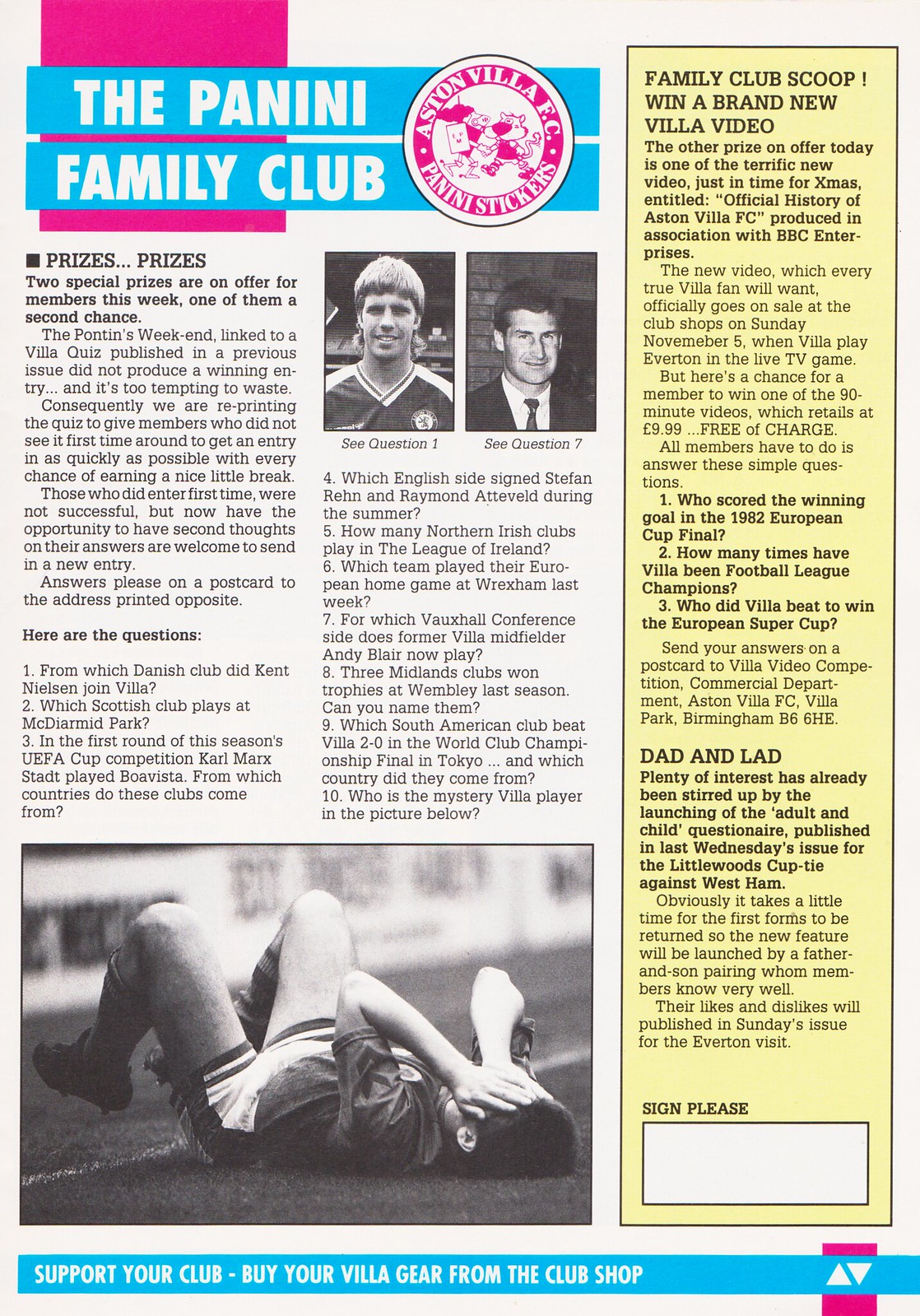This detailed image appears to be a page out of a sports magazine, dedicated to the Panini Family Club, specifically celebrating the Aston Villa football team. At the top of the page, there is a bold title that reads "The Panini Family Club" in white capital letters set against a light blue background. Behind the title is a fuchsia square, and adjacent is the club's circular logo, featuring white and fuchsia colors with the words "Aston Villa EC Panini stickers."

Directly below the title, two photographs are prominently displayed. The first image captures a man in a sports uniform, with the caption "see question one" underneath. The second photo shows a man in a suit and tie, with "see question seven" printed below his image. The page contains an article split into two columns, discussing various aspects of the club, including a special mention of "prizes, prizes – two special prizes are on offer for members this week, one of them being a second chance.” This section highlights a reprint of a previous quiz for members who missed it, encouraging quick participation for a chance to win a break.

On the page's right side, there is a vertical yellow sidebar with more information about the club. This box, detailed with black type on a beige background, features a headline "Family Club Scoop – Win a brand new Villa video.” As the article continues, at the bottom part of the page, a black and white photograph shows a soccer player lying on the field, covering his face with his hands, associated with the headline "Dad and Lad." Near the bottom, a thin blue banner encourages readers to "Support your club, buy your Villa gear from the club shop." The overall layout, with its tan, pink, purple, blue, white, gray, and yellow colors, confirms it as a vibrant magazine page dedicated to avid fans of the Aston Villa football club.